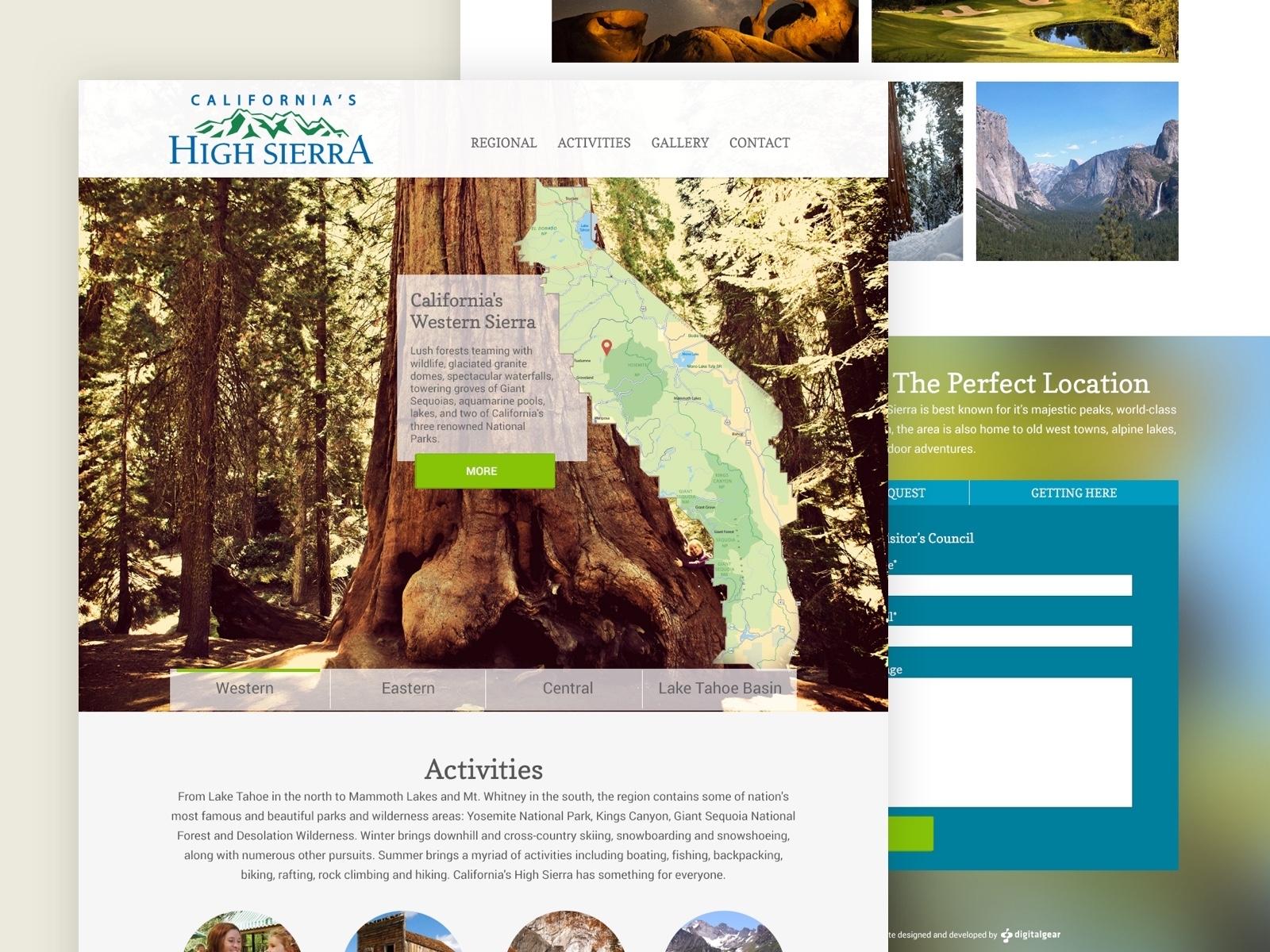Screenshot Description:

The screenshot captures a detailed webpage, set against a cream-colored, tan background. Multiple images and textual elements are arranged across the interface. On the left-hand side, there's a prominent headline in dark blue text reading "Californias," accompanied by a dark green, white-rimmed silhouette of a mountain range, and a bold, blue title, "High Sierra."

To the right, a light gray bordered pop-up window appears, showcasing several dark gray, all-cap buttons: "REGIONAL," "ACTIVITIES," "GALLERY," and "CONTACT." Below it, a large, dark brown and red redwood tree is featured with surrounding trees bearing yellow and green foliage. An opaque rectangle superimposed on the tree displays text describing California's Western Sierra: "California's Western Sierra is a lush forest teeming with wildlife, glaciated giant granite domes, spectacular waterfalls, towering groves of giant sequoias, aquamarine pools, lakes, and two of California's three renowned national parks." At the center of this section, a lime green button marked "MORE" in white text invites further exploration.

Near the bottom of the page, several light gray, semi-transparent tabs read "WESTERN," "EASTERN," "CENTRAL," and "TAHOE BASIN" in dark gray text. Another slightly off-white rectangle with gray and possibly blue highlights centers bold black text stating "ACTIVITIES." Regular black text below elaborates on California's High Sierra, mentioning destinations and activities: "From Lake Tahoe in the north to Mammoth Lakes and Mt. Whitney in the south, the region contains some of the nation’s most famous and beautiful parks and wilderness areas... Yosemite National Park, Kings Canyon, and Sequoia National Forest and Desolation Wilderness. Winter brings downhill and cross-country skiing, snowboarding, and snowshoeing, along with numerous other pursuits. Summer brings a myriad of activities including boating, fishing, backpacking, biking, rafting, rock climbing, and hiking. California's High Sierra has something for everyone."

At the bottom, various images depict scenes: two women beside a shack amidst green trees, the edge of an old brown and tan building against a dark blue cloudy sky, an arch resembling a cavern entrance in tan, brown, and gray, and a snow-capped dark gray mountain range under a blue sky. Another pop-up window with bold white text reads "THE PERFECT LOCATION." Beneath it, partially cut-off white text implies Sierra's acclaim for majestic parks, world-class attractions, old west towns, alpine lakes, and adventure opportunities. A dark blue rectangle with two visible clickable buttons labeled "QUEST" and "GETTING HERE" in white text appears, alongside some text mentioning a council and a submission button obscured by a large rectangle.